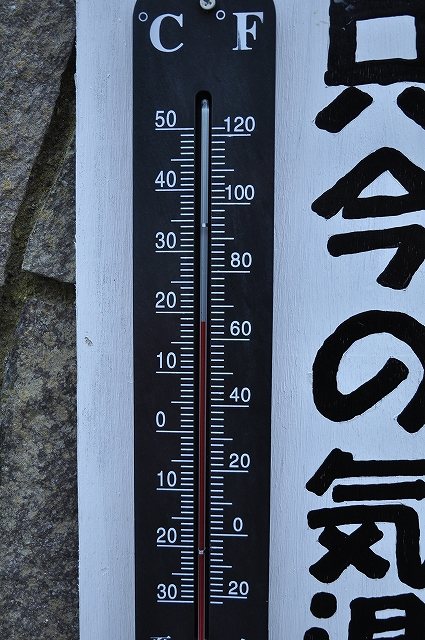The image features a thermometer placed on outdoor pavement, captured with great detail. On the left side, part of the background reveals three tiles in varying shades of brown, ranging from light to dark. Between these tiles, there is grout that appears to be a mix of greenish and dark brown hues. 

The thermometer itself is mounted on a white-painted wooden board. The thermometer is a black vertical strip against the white background, with white numerical markings on both sides. The left side of the thermometer measures temperatures in Celsius, starting at -30, and increasing through -20, -10, 0, 10, 20, 30, 40, up to 50 degrees Celsius, with smaller tick marks in between.

On the right side, the thermometer measures temperatures in Fahrenheit, starting from -20, progressing through 0, and climbing up to 120 degrees Fahrenheit. To the extreme right of the thermometer, there is black text written in what appears to be Chinese characters, adding an additional international element to the image.